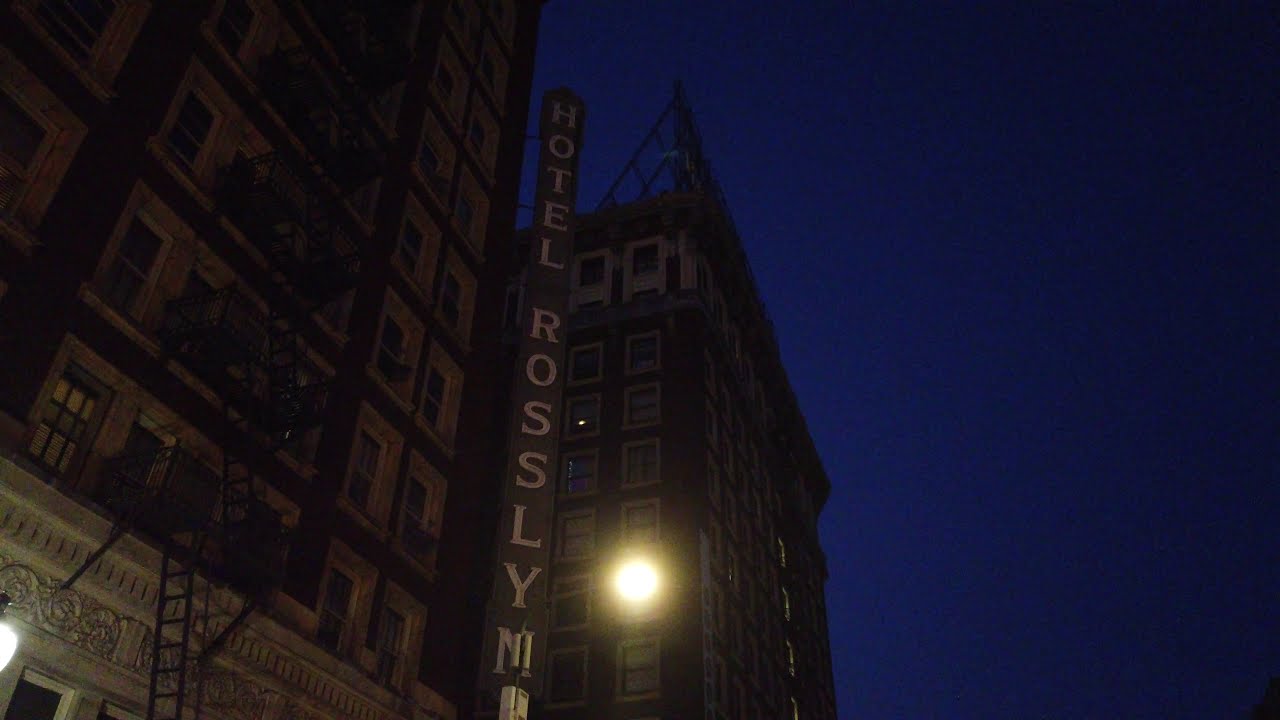The photograph captures a nighttime scene with two prominent, older brick buildings towering upwards against a deep royal blue, clear sky. The image looks up from street level, giving a dramatic perspective. On the right building, there is a bright, round streetlight shining in front of one of the windows, casting a white light that fades into a yellow orb. The center and left sides of the photograph display a building with numerous small windows and a black metal fire escape running vertically along its side. A notable feature is a vertical sign between the two buildings with white, vertically aligned lettering that reads "Hotel Rosslyn," although the last letter is somewhat obscured by a streetlamp post. The evening setting highlights the buildings' detailed architecture and the eerie upside-down "Hotel Rosslyn" words on a board attached to one building, enhancing the photo's atmospheric depth. The overall scene evokes a sense of historic charm and urban mystique.